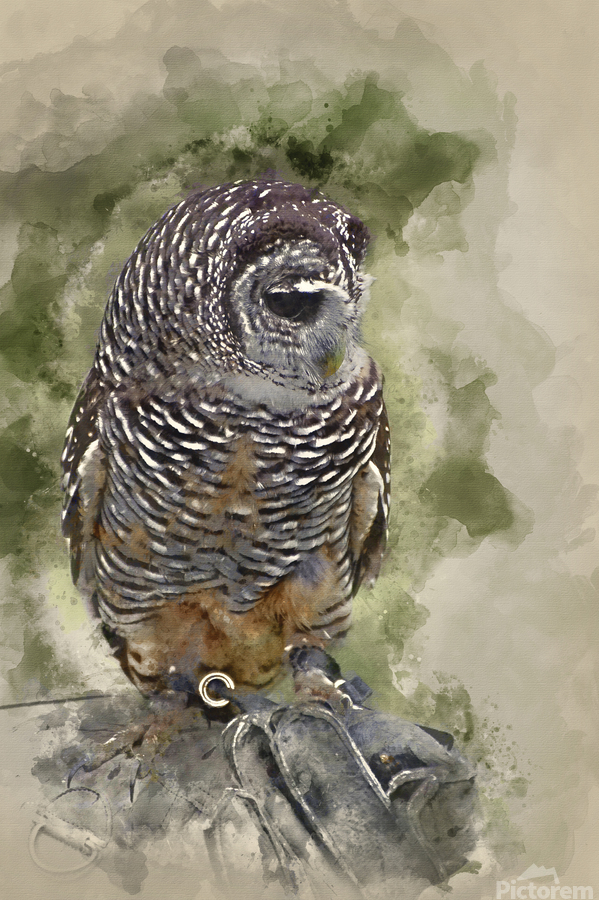This watercolor painting features a striking owl, predominantly brown with a mix of light and dark brown feathers, and accented by white and yellowish-brown hues. The owl's dark black eyes and yellow beak stand out against its whitish face, giving it a piercing look. The bird is positioned with its wings close to its body, perched atop a complex array of what appears to be leather straps and metal, including a visible ring or buckle around its foot, suggesting it may be in captivity or used by a trainer. Its black talons grip the straps, adding to the intricate detail at the lower part of the image. The background transitions from light tan to varying shades of sage green, with some beige smudges enhancing the natural feel. The composition is signed "Pictorem" in white text in the lower right corner, adding a professional touch to this evocative artwork.